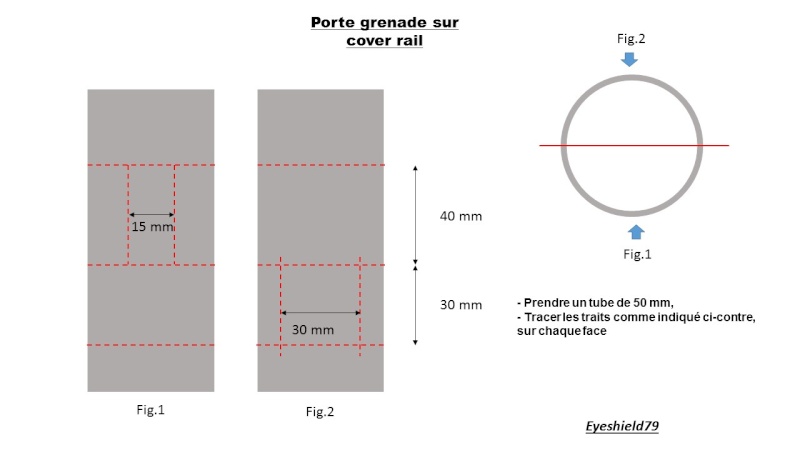The diagram is labeled in French and features several detailed components on a white background. To the top, black text reads "Porte Granade Sur Cover Rail." On the left side, there are two vertical gray rectangles, each with red dotted lines and measurements in millimeters. The first rectangle is marked "figure 1" with a label of 15 mm, and the second is marked "figure 2" with a label of 30 mm. Both figures have black text labels with millimeter measurements and are accompanied by blue arrows pointing towards another section on the right. This section features a gray circle divided horizontally by a red line into two semicircles, with "figure 2" on top and "figure 1" at the bottom. Beneath the circle are further French text labels: "Pendre Un Tube De 50mm" and "Treseles Traits Como Indique Si Contres Sur Chaque Face." At the bottom right, underlined text reads "iShield 79."